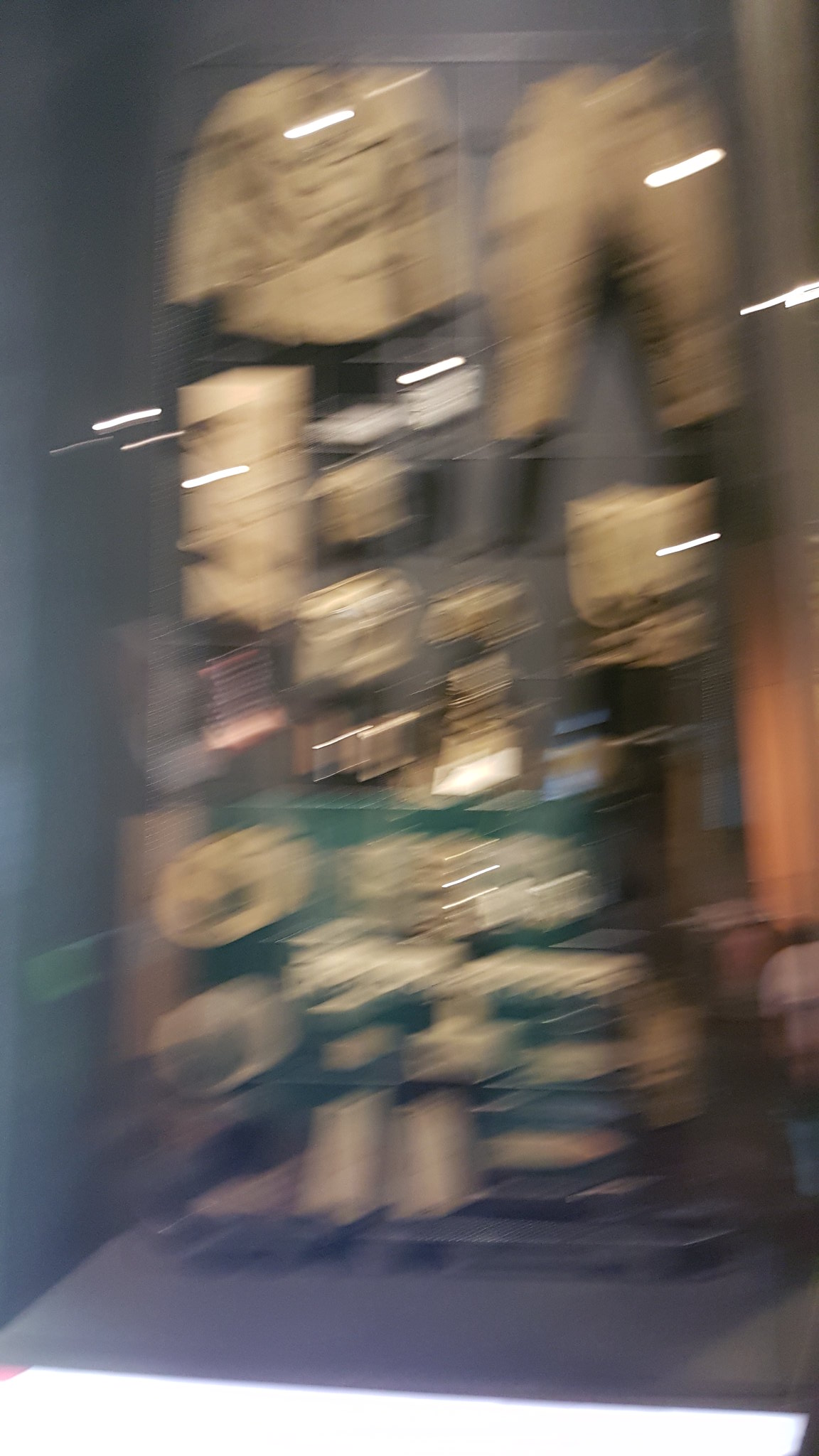The image, in a portrait format and highly blurred due to significant motion, depicts a retail store for apparel with a gray background. The store features a display area that is twice the height of a person, showcasing various items of camo clothing. In the upper left corner, a camo jacket is visible, while camo pants occupy the upper right. Below these, a vertical camo rectangle, possibly a bag, and three smaller squarish items are present. On the right side, there's another vertical camo rectangle. A green cube display below features several straw hats. The presence of fluorescent ceiling lights and motion lines enhance the impression of rapid movement, likened to a warp speed effect, adding to the image’s overall distortion and dynamic feel.